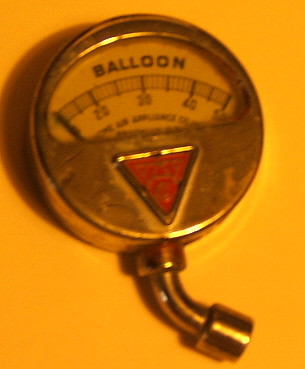An indoor, color close-up photograph features a chrome circular object against an orange background. The centerpiece of the object is an oval opening located on its upper half, containing a white-faced gauge with black markings ranging from 0 to 50, reminiscent of a tachometer or speedometer in a car. Above the gauge, the word "Balloon" is prominently displayed in black letters. Below the gauge, the chrome surface is adorned with a red triangle, although the text within the triangle is indistinguishable. 

The triangle points downward, leading to a chrome elbow fitting that bends gently to the lower right corner, approximately at a 60-degree angle. The object appears used and dirty, with noticeable pitting on the chrome surface, especially around the gauge opening. The image is slightly out of focus, with lighting emanating from the lower right, casting shadows towards the upper left. The overall condition and design suggest that this gauge is related to some aspect of balloon operation. No additional words or text are present in the image.